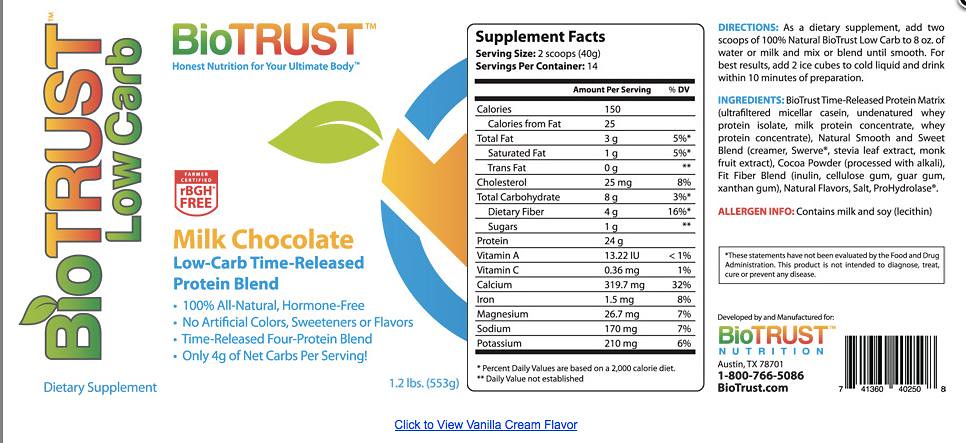Detailed Caption:
The product label for "BioTrust Low Carb Honest Nutrition for Your Ultimate Body" introduces a dietary supplement recognized for its milk chocolate flavor and low-carb, time-released protein blend. Originating from Austin, Texas, the label specifies that the product is designed as a protein drink. Consumers are instructed to utilize the supplement by adding two scoops of the 100% natural BioTrust powder to 8 ounces of water or milk, blending it thoroughly before consumption. The label features comprehensive health and nutritional information, including supplement facts, and ingredient details. The overall aesthetic of the label is quite understated, dominated by a light blue color for most of the text and accented with fluorescent green for the words "Bio" and "Low Carb." The writing is clear and primarily in black, offering an uncluttered and straightforward presentation.